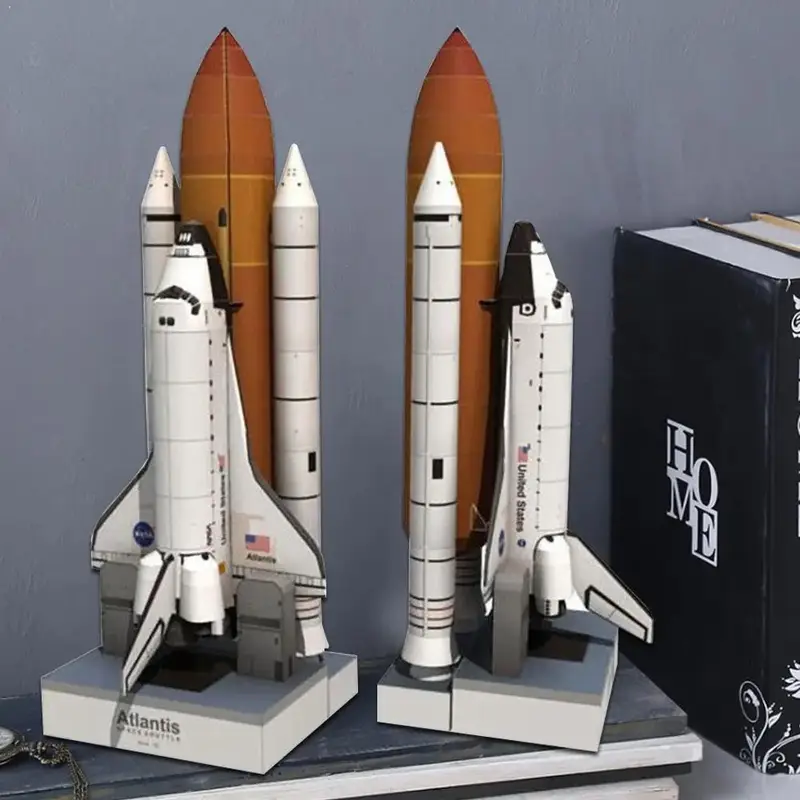The image showcases two detailed models of NASA Space Shuttles, prominently featuring the Shuttle Atlantis. Both models are positioned upright, attached to the familiar orange central fuel tank and adjacent white rocket boosters as if poised for launch. They exhibit the distinctive design elements of real shuttles, with black underbellies, wings, and tails. Each model displays a "United States" label along with an American flag, and both have a black tip. These miniature replicas are mounted on gray brackets for stability and rest on a table with a gray top and white bottom. The backdrop includes a gray wall and a bookshelf to the right, where a black book with "HOME" written on its spine, arranged into two lines (H-O, M-E), stands alongside other stacked books. The models function as bookends or decorative pieces, adding a touch of space exploration to the scene.